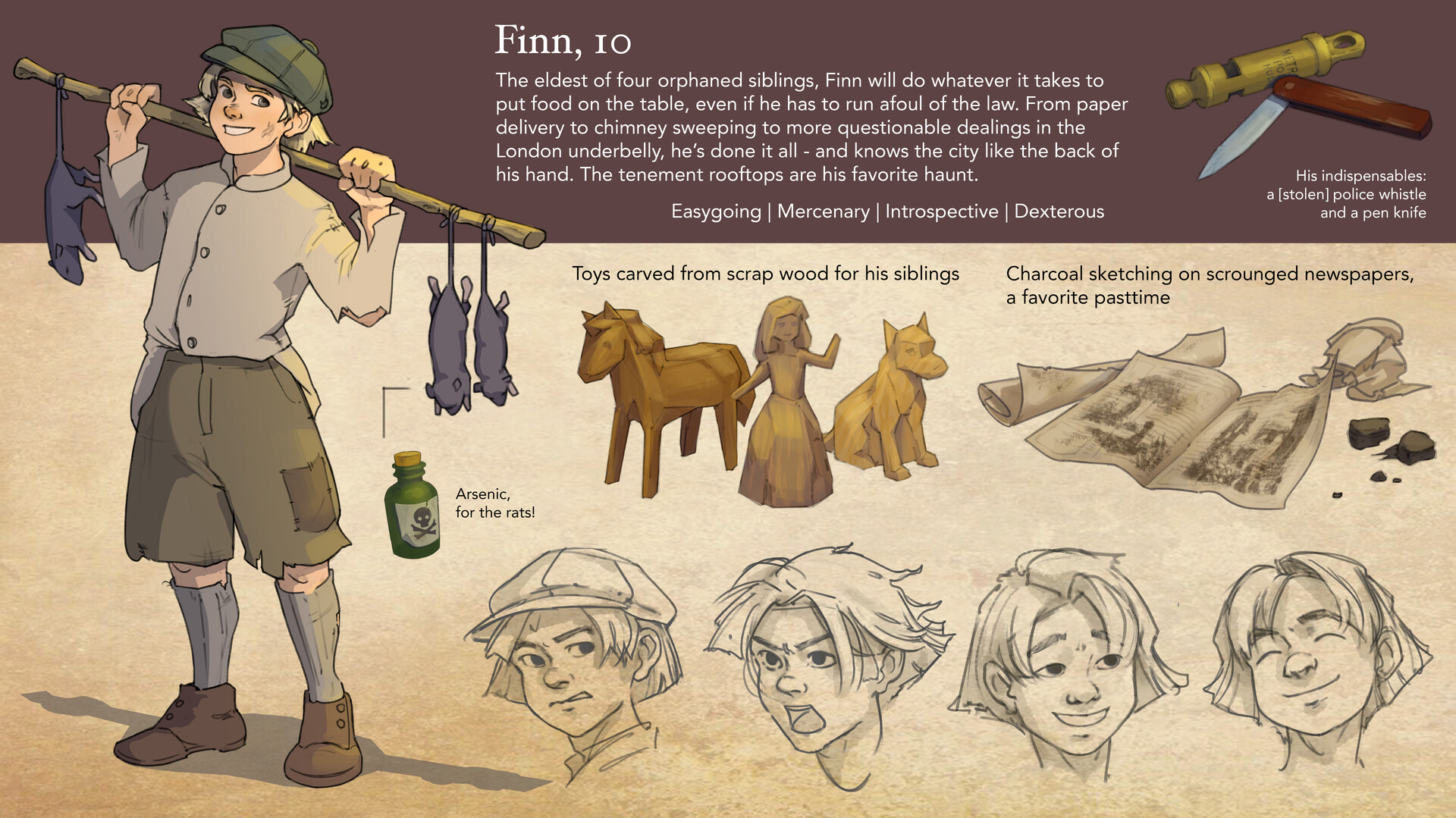This detailed concept art image presents Finn, a ten-year-old character who is the eldest of four orphaned siblings. Determined to provide for his family, Finn takes on any job necessary, from paper delivery and chimney sweeping to more dubious activities in London's underbelly. The image's top section contains a descriptive paragraph about Finn, highlighting his extensive knowledge of the city and his favorite haunt—the tenement rooftops. The text continues to describe him as easygoing, mercenary, introspective, and dexterous, with his indispensable items being a pen knife and a stolen police whistle.

On the left side of the image is a full-body illustration of Finn, dressed in a green cap, a long-sleeved gray shirt, and gray trousers that fall to his knees, complemented by brown shoes and gray socks. He is holding a long quarterstaff over his shoulder, from which three dead rats hang by their tails, and is depicted with a smile. Below this, the image displays four different expressions of Finn's face—confusion, anger, happiness, and satisfaction.

The image also showcases several items related to Finn: toys carved from scrap wood intended for his siblings, and a charcoal sketch on scrounged newspapers—a reflection of his favorite pastime. Additionally, there is a green bottle of arsenic labeled "for the rats" featuring a skull and crossbones. In the upper right-hand corner, the image highlights a pen knife and a stolen police whistle, central to Finn's resourcefulness and survival in the harsh streets of London. The background transitions from dark brown at the top to light brown at the bottom, bringing a warm yet somber tone to the overall depiction.